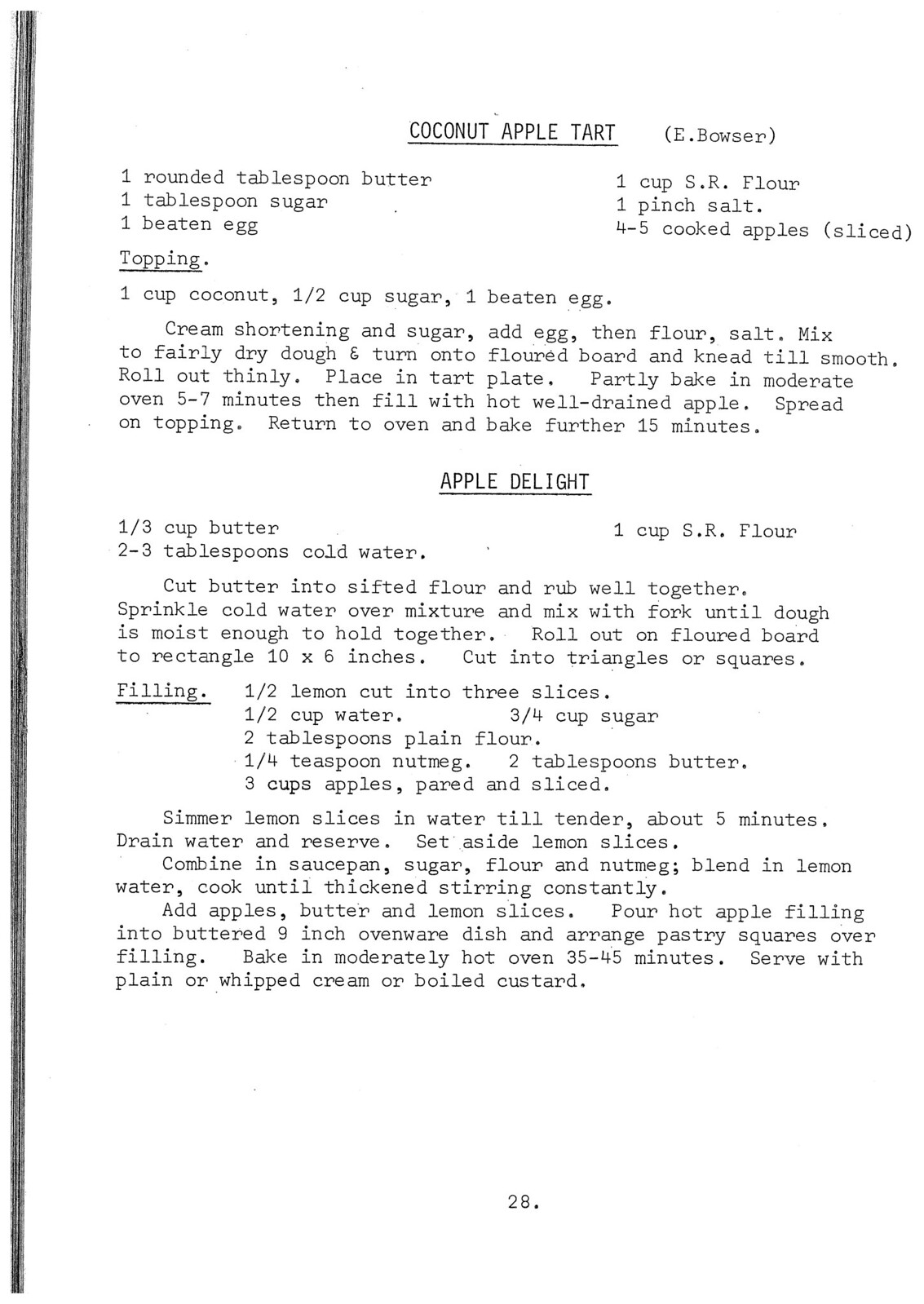This image depicts an old sheet of paper, specifically page 28 of a larger recipe book. The page includes two typed recipes labeled "Coconut Apple Tart" and "Apple Delight," both titles underlined in black and written in uppercase letters. At the top, it mentions "Coconut Apple Tart" followed by "eBowser" in parentheses, likely indicating the recipe's creator. The document is marked by a vertical black line running down the far left side, possibly a scan mark or margin. 

The "Coconut Apple Tart" recipe lists ingredients such as one rounded tablespoon of butter, one tablespoon of sugar, and one beaten egg, along with detailed instructions: "Cream shortening and sugar, add egg and flour, salt. Mix to a fairly dry dough and knead until smooth. Roll out thinly, place in tart plate, and partly bake in a moderate oven for 5 to 7 minutes. Then fill with well-drained hot apple, spread on topping, and return to the oven to bake for an additional 15 minutes."

Below it, the "Apple Delight" recipe includes ingredients like one-third cup of butter, two to three tablespoons of cold water, and one cup of SR flour. Instructions follow similarly structured.

Both recipes also include sections on making their respective toppings and fillings. The overall appearance of the document, with its typewriter text and vintage condition, suggests that it is part of an old-fashioned cookbook.